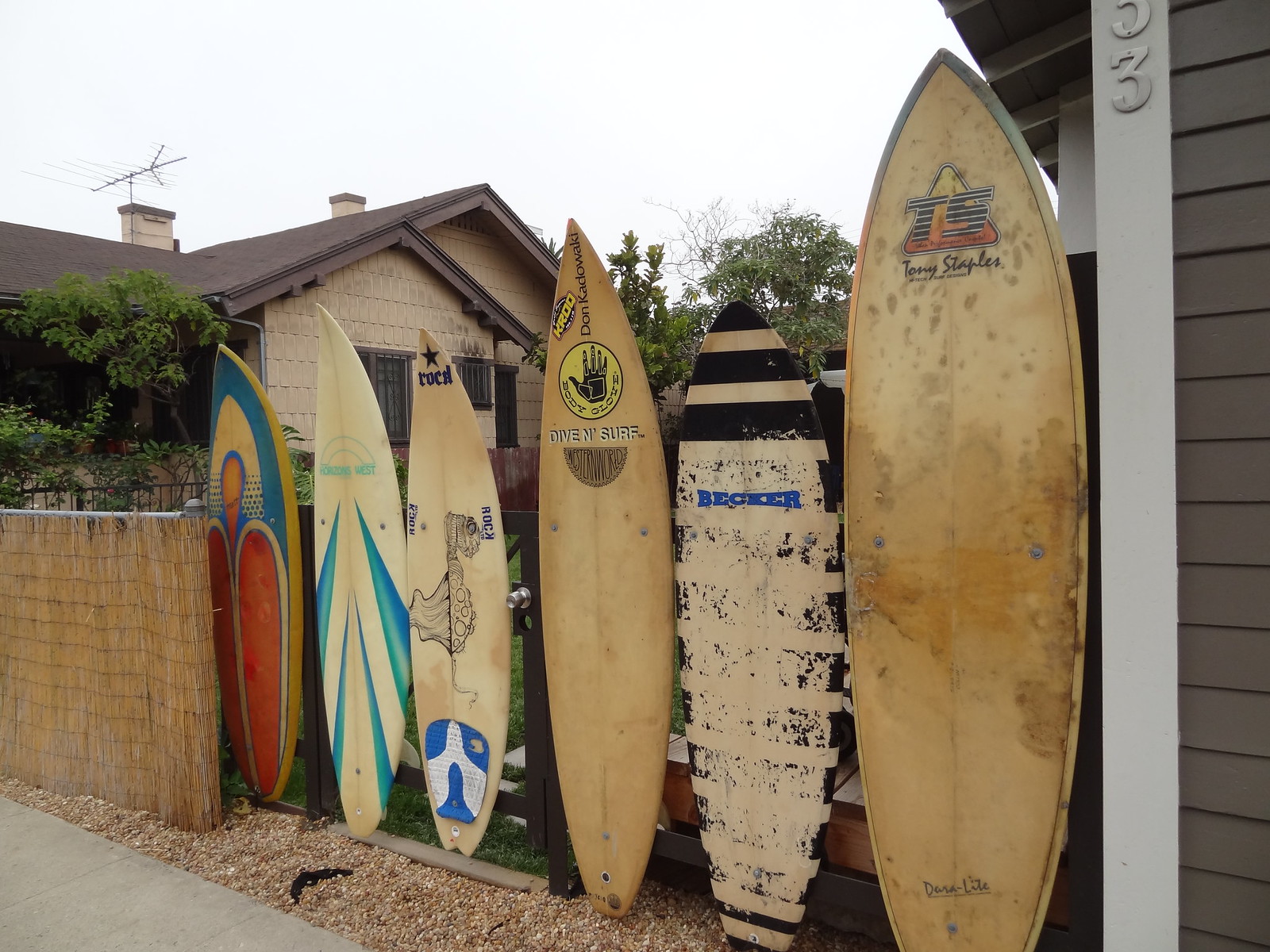The photograph depicts a unique fence made of six old wooden surfboards positioned along the side of a house, visible from the street. These surfboards, with visible wear and tear, vary in length and design, showcasing their age and usage. The boards range from natural wood hues to vibrant designs; the leftmost surfboard features red, orange, and blue patterns, while the next one displays teal and blue triangles. The third surfboard has an indistinguishable black image and a blue and white logo near the bottom. The fourth bears a Body Glove logo, and the fifth, branded Becker, shows remnants of black stripes along its worn surface. The sixth and most prominent board has a TS logo at the top, accompanied by unreadable script.

These surfboards are integrated into an actual gate and fence: a brick wall transitions into a regular wicker-like fence, ending where the surfboards start. Behind this quirky fence, a handle reveals the presence of a gate that swings open with the surfboards attached. The backdrop includes a tan house with a brown roof, adorned with a TV antenna. Additionally, a small part of another house is visible, characterized by brown walls and grayish trim, with only the last house number "3" discernible. The daytime scene is complemented by trees in the background and river stones lining the edge of the property.